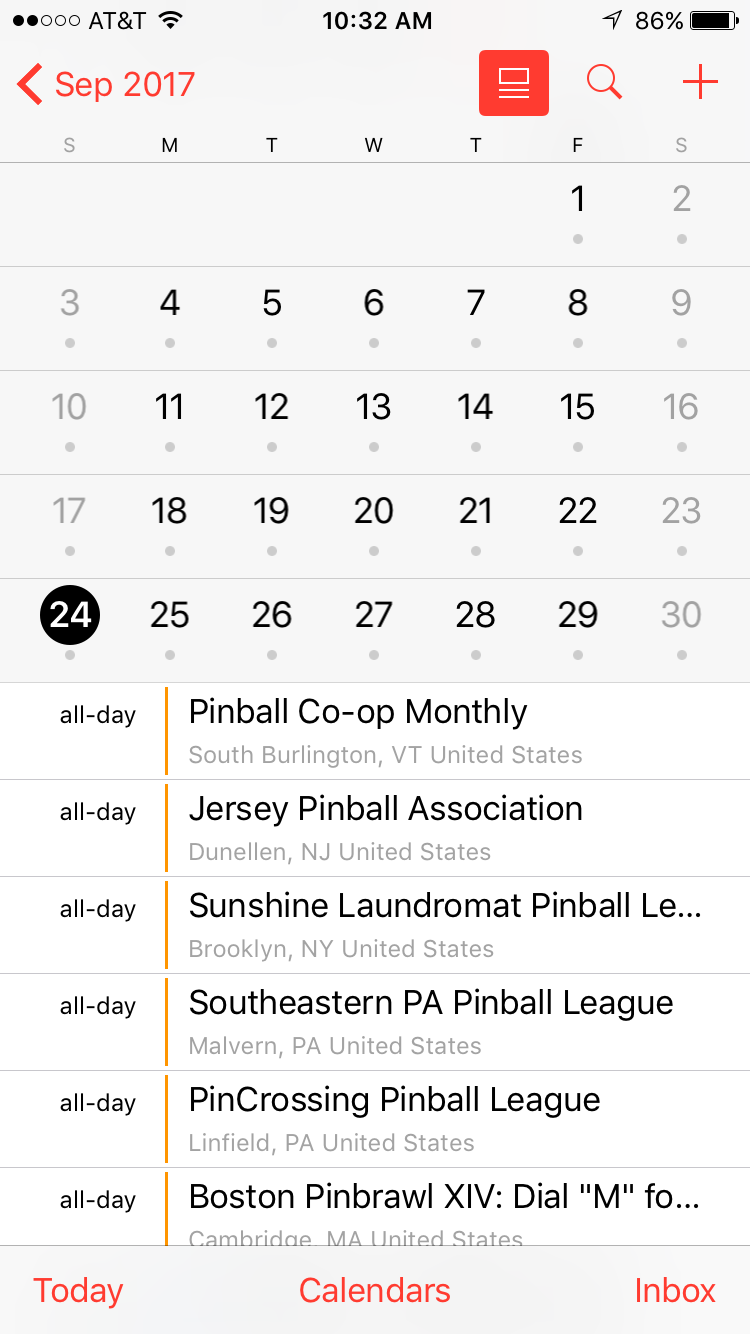The image depicts a digital calendar displayed on a cell phone. At the top of the screen, the status bar is visible, showing the signal strength, Wi-Fi connectivity, current time, and battery level. The calendar is set to September 2017, with the 24th day prominently highlighted. Below the calendar grid, a detailed list of events scheduled for that day are displayed, each marked as "All Day" events. 

The listed events are:
- Pinball Co-op Monthly in South Burlington, Vermont, United States
- Jersey Pinball Association in Dunnellan, New Jersey, United States
- Sunshine Laundromat Pinball League in Brooklyn, New York, United States
- Southeastern Pennsylvania Pinball League in Malvern, Pennsylvania, United States
- Pincrossing Pinball League in Linfield, Pennsylvania, United States
- Boston Pinball's "Pinbrawl 14, Dial M4..." event in Cambridge, Massachusetts, United States 

Each event spans the entire day, highlighting various pinball leagues and tournaments happening across different locations in the United States.